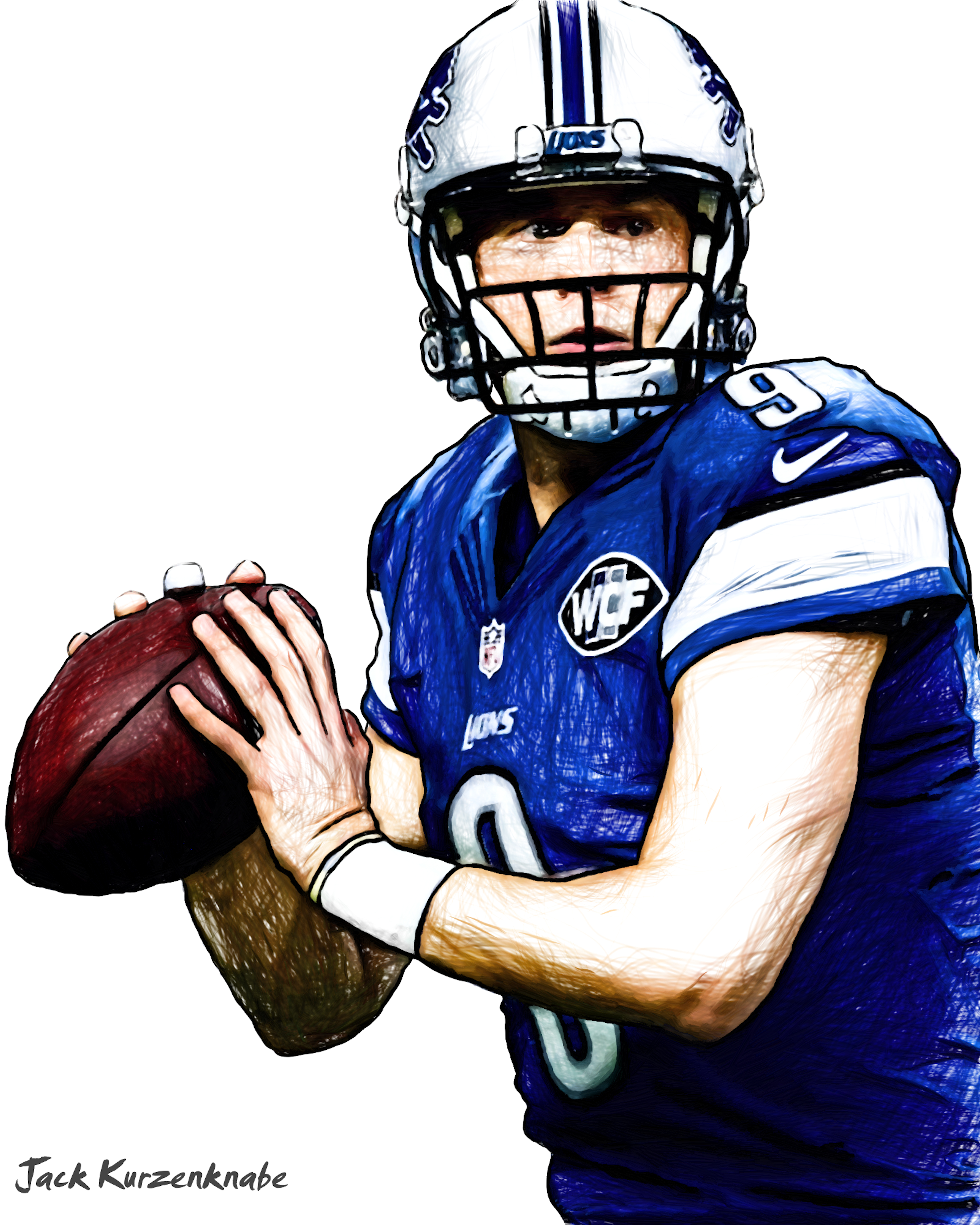The image is a detailed, heavily filtered photograph that resembles a hand-drawn depiction of an NFL quarterback, presumably Matthew Stafford. The football player is captured mid-throw, visible from the waist up, facing slightly right with his eyes while his torso remains front-facing. He wears a dark blue jersey featuring white stripes on the sleeves, white numbers '9' on the shoulder pads and front, and 'Lions' text on the chest area. A silver helmet with blue stripes and logos, indicative of the Detroit Lions, protects his head. His left wrist is adorned with a white wristband, while his right hand grips a brown football, partially obscured by his body. The background is stark white, accentuating the player. Notably, the artwork includes small black text in the bottom left corner reading "Jack Curzon Gnabey," highlighting the artist's signature. The image, while clearly created with digital filters, effectively simulates a hand-drawn style.